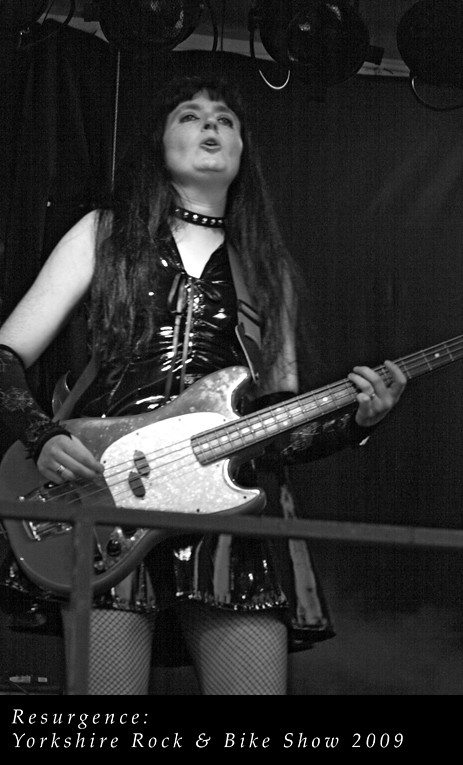This black and white photo captures a female performer on stage with an electric guitar, mid-performance. She has long dark hair and is wearing a black leather or pleather vest and a matching short skirt. Adding to her edgy look are fishnet tights and a spiked black leather choker around her neck. She sings into a microphone while facing the camera, although her gaze does not meet the lens directly. At the bottom of the image, there is a caption that reads: "Resurgence: Yorkshire Rock and Bike Show 2009".